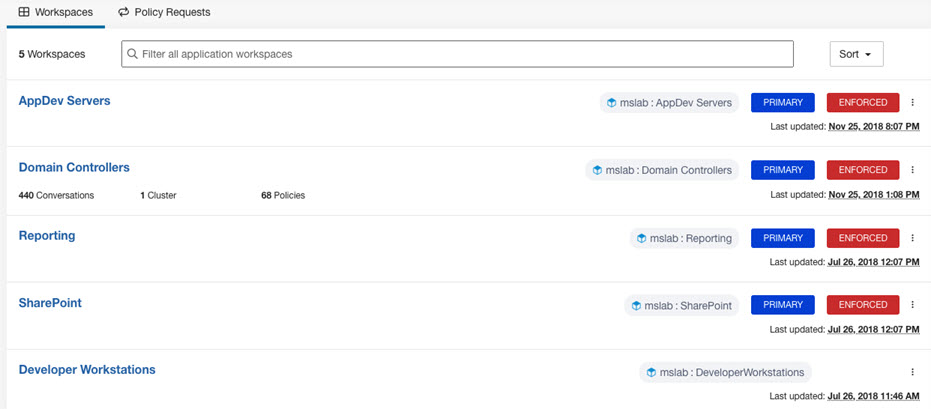Here is the cleaned up and detailed caption for the image:

---

The image depicts a user interface from a Workspace website. At the top left corner, there is a label "Workspaces" which is underlined in blue. To its right, another label reads "Policy Requests," both of which are set against a gray bar background.

Below this gray bar, a highlighted section indicates five workspaces, accompanied by a data field labeled "Filter All Application Workspaces," outlined in gray. Beneath this, a blue header reads "App Developer Servers," followed by a horizontal gray line.

On the right-hand side of this section, there is an entry for "MS Lab App DDev Service" showcasing a blue button labeled "Primary" and a red button labeled "Enforced." The last update for this entry is noted as November 25, 2018, at 8:07 p.m.

Further below, the section titled "Domain Controllers" indicates 440 conversions, one cluster, and 68 policies. To the right of this, another entry shows "MS Lab Domain Controllers," also featuring the blue "Primary" and red "Enforced" buttons. This was last updated on November 25, 2018, at 1:08 p.m.

The subsequent section is labeled "Reporting," with a corresponding entry "MS Lab Reporting" on its right, displaying the familiar blue "Primary" and red "Enforced" buttons. The last update for this entry was on July 26, 2018, at 12:07 p.m.

Finally, the last section titled "SharePoint" includes an entry for "MS Lab SharePoint," also accompanied by the blue "Primary" and red "Enforced" buttons, last updated on July 26, 2018, at 12:07 p.m.

---

This caption provides a meticulous and comprehensive description of each element and section visible in the image.